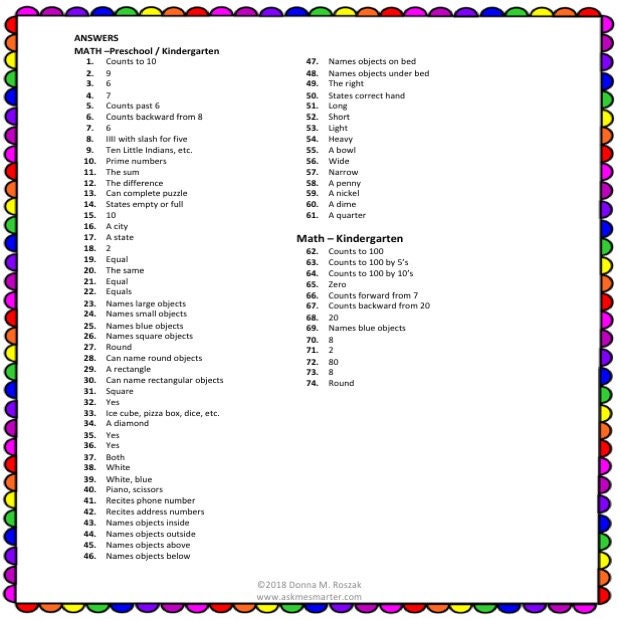The image displays an extensive, detailed list numbered sequentially from 1 to 74. The list is organized into three primary sections, each containing multiple items with varying descriptions.

In the first section, the numbers run from 1 to 46 on the left-hand side. Here is a breakdown of some key items from the list:
1. Counts from 1 to 10.
2. Counts to 9.
3. Counts to 6.
4. Counts to 7.
5. Counts past 6.
6. Counts backwards from 8.
7. Counts to 6.
8. Slash for 5.
9. Ten Little Indians (descriptive phrase).
10. Prime numbers.
11. The sum.
12. The difference.
13. Can complete puzzles.
14. States (empty or full).
15. Ten.
16. A city.
17. A state.
18. Two.
19. Equal.
20. The same.
21. Equal.
22. Equal.
23. Names large objects.
24. Names small objects.
25. Names blue objects.
26. Names square objects.
27. Names round objects.
28. Can name round objects.
29. Names rectangular shapes.
30. Can name rectangular objects.
31. Square.
32. Yes.
33. Objects such as ice cubes, pizza boxes, dice, etc.
34. Diamond.
35. Yes.
36. Yes.
37. Both.
38. White.
39. White and blue.
40. Piano and scissors.
41. Recites phone number.
42. Recites address number.
43. Names objects inside.
44. Names objects outside.
45. Names objects above.
46. Names objects below.

Transitioning to the second section, the numbers 47 to 61 are also detailed items:
47. Names objects on the bed.
48. Names objects under the bed.
49. The right.
50. States correct hand.
51. Long.
52. Short.
53. Light.
54. Heavy.
55. A bowl.
56. Wide.
57. Narrow.
58. A penny.
59. A nickel.
60. A dime.
61. A quarter.

The final section, numbered 62 to 74, is titled "Math, Kindergarten":
62. Counts to 100.
63. Counts to 100 by fives.
64. Counts to 100 by tens.
65. Zero.
66. Counts forward from seven.
67. Counts backwards from 20.
68. Twenty.
69. Names blue objects.
70.
71. Two.
72. Eighty.
73. Eight.
74. Round objects.

The list is set against a white background adorned with a decorative border consisting of half circles in various colors, including purple, pink, green, yellow, orange, and red. This colorful border runs along the top, bottom, left, and right edges of the image.

At the very bottom center, the image includes a copyright notice: "Copyright 2018 Donna M. Rozak, www.askmesmarter.com."